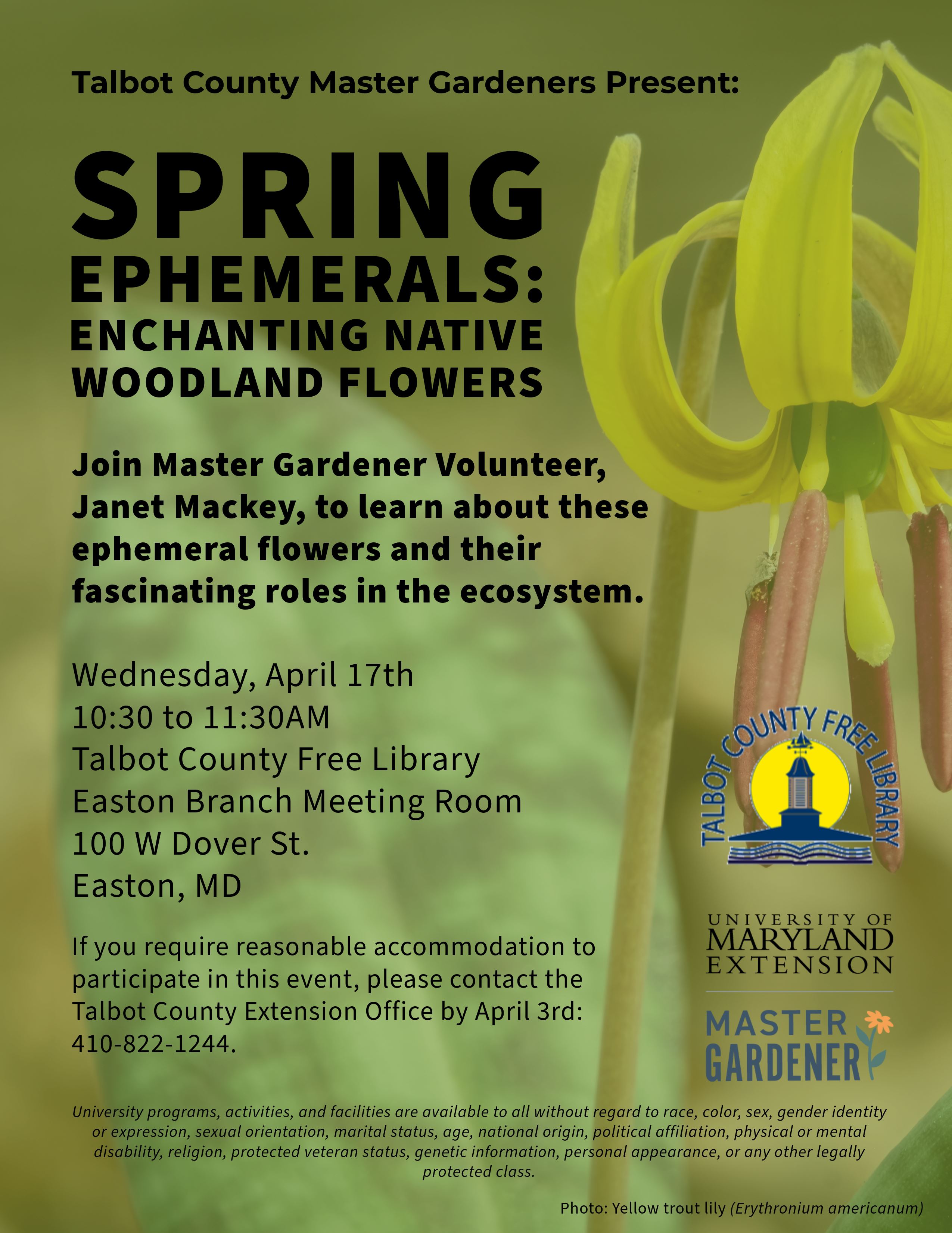The flyer features a pea green background and prominently displays a detailed illustration of a yellow daffodil-like flower with a long, skinny green stem and red rectangular extensions on its green bud. The top of the flower droops downward. At the top of the flyer, in bold black text, it reads, "Talbot County Master Gardeners Presents," followed by larger bold letters announcing, "Spring Ephemerals: Enchanting Native Woodland Flowers." Beneath this title, a subtitle invites readers to "Join Master Gardener volunteer Janet Mackey to learn about these ephemeral flowers and their fascinating roles in the ecosystem." 

Further down, the flyer lists event specifics: "Wednesday, April 17th, from 10:30 to 11:30 a.m. at Talbot County Free Library Eastern Branch Meeting Room, 100 W. Dover Street, Easton, MD." It also notes that individuals requiring accommodations should contact the Talbot County Extension Office by April 3rd at 410-822-1244. 

On the right side of the flyer, there are logos for the Talbot County Free Library, showcasing a lighthouse with a sun behind it, and the University of Maryland Extension Master Gardener. Additional event and contact information is provided in black text at the bottom of the page.